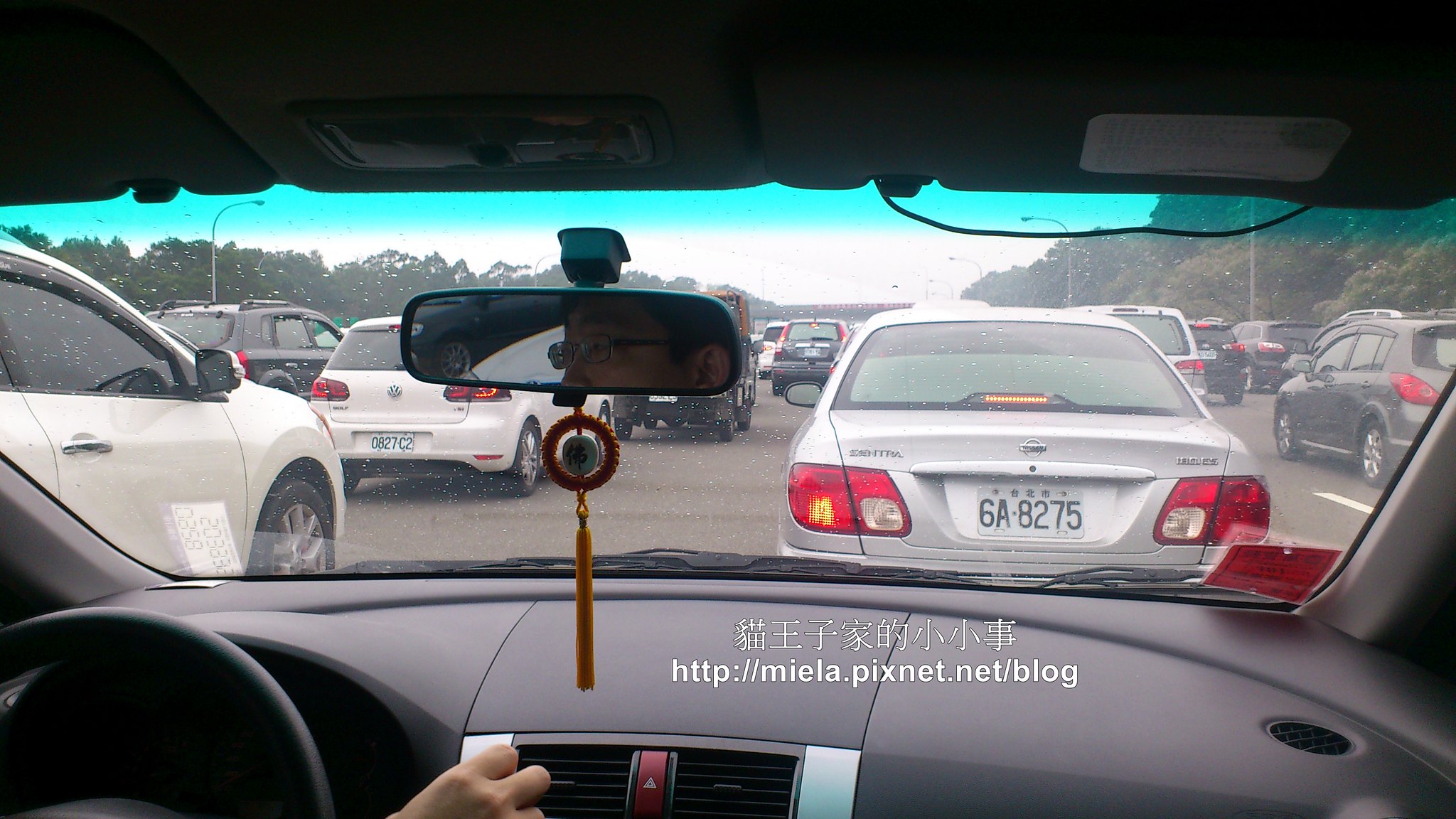A detailed photograph captures an interior view from within a car, taken from the perspective of the passenger seat looking towards the driver. The driver's right hand, partially visible, is reaching out to adjust an air vent on the sleek, black plastic dashboard. Reflected in the rearview mirror, the driver's focused face can be seen. A vibrant red tassel dangles from the rearview mirror, adding a splash of color to the scene. Raindrops delicately dot the windshield, suggesting a recent or ongoing drizzle. Outside the car, a busy roadway stretches ahead, filled with an assortment of vehicles in shades of white, gray, and black, creating a monochromatic urban palette.